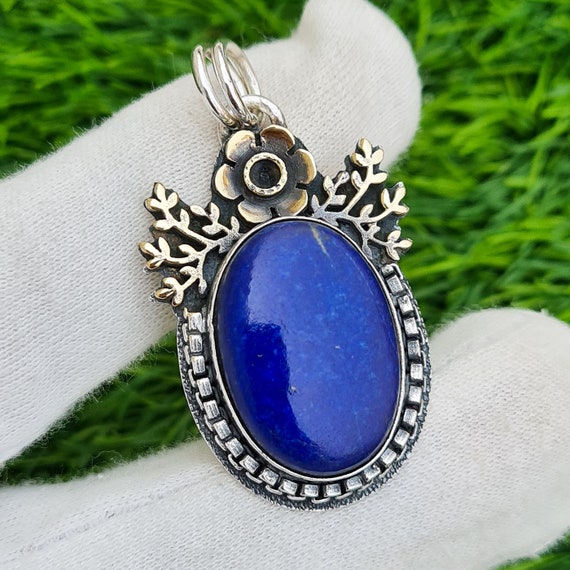The photograph captures a detailed shot of a piece of jewelry, likely the main focal point of a necklace. This blue jewel, possibly an opal with lighter blue flecks, is encased in a somewhat tarnished silver setting. The centerpiece of the jewelry is a prominent oval-shaped blue stone. At the top of the stone, there's a delicate silver flower with intricately carved leaves extending to the sides. This floral arrangement is possibly missing a tiny jewel. The jewelry hangs from a double ring, suggesting it is designed to be attached to a necklace. The piece is held delicately by a gloved mannequin hand, and the background features a contrasting vibrant green grass or shredded paper, enhancing the elegance of the jewel against the white glove.